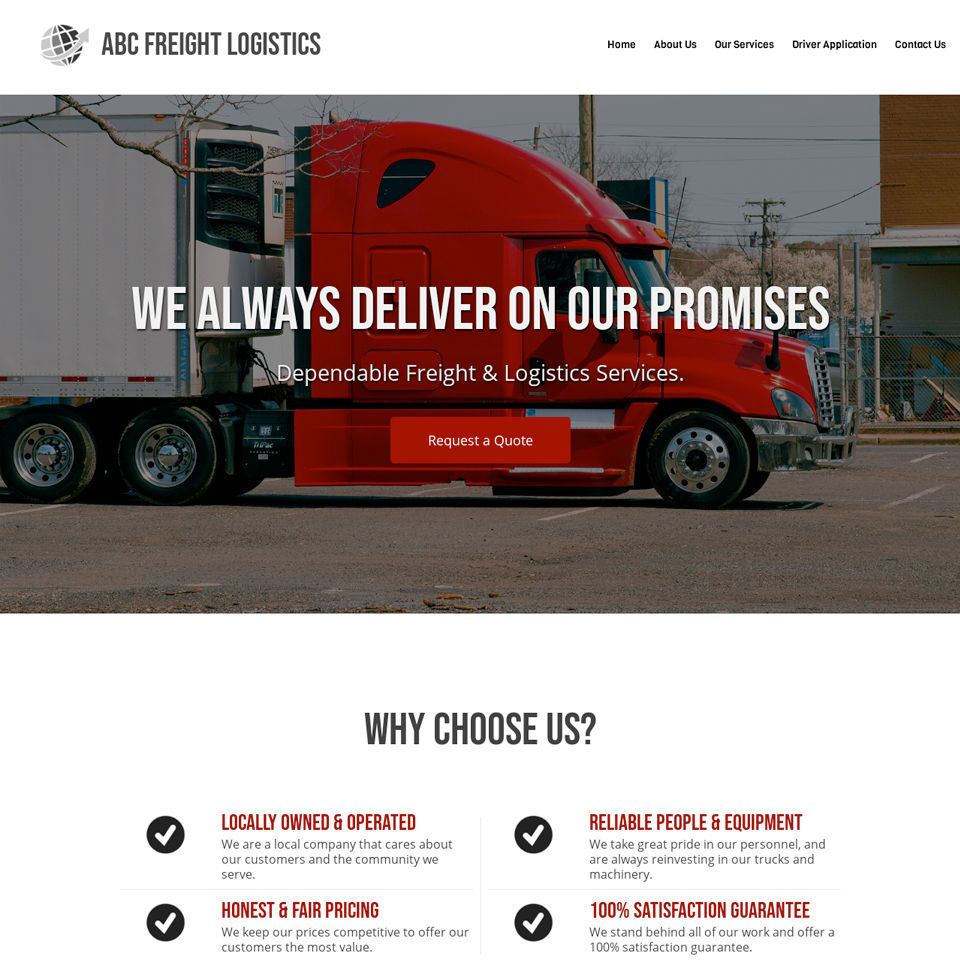A screenshot of the ABC Freight Logistics website showcasing their homepage. The company's logo features a globe icon with a swooping arrow next to the text. In the upper-right corner of the page, there are navigation links for Home, About Us, Our Services, Driver Application, and Contact Us. The hero section of the page displays a striking image of a red 18-wheeler cab with a white trailer, positioned in a parking lot amidst industrial elements such as telephone poles and what appear to be generators or buildings in the background. This image is dimmed by a 50% graded black overlay, and across the top, bold white capital letters proclaim, "We always deliver on our promises." Below this statement, in large text, are the words, "Dependable Freight and Logistics Services," and a prominent red call-to-action button labeled "Request a Quote."

Beneath this hero section, a white background features a centered heading in black text that reads, "Why Choose Us?" Four benefits are listed beneath, each accompanied by a black circle with a white check mark. The benefits include:

1. **Locally Owned and Operated** - Emphasizing the local roots of the business.
2. **Honest and Fair Pricing** - Highlighting their commitment to transparent and reasonable prices.
3. **Reliable People and Equipment** - Ensuring dependable service and trustworthy equipment.
4. **100% Satisfaction Guarantee** - Accompanied by a smaller text that reads, “We stand behind all of our work and offer 100% Satisfaction Guarantee,” highlighting their confidence in their services.

This detailed layout underscores the company's pledge to reliability and customer satisfaction.